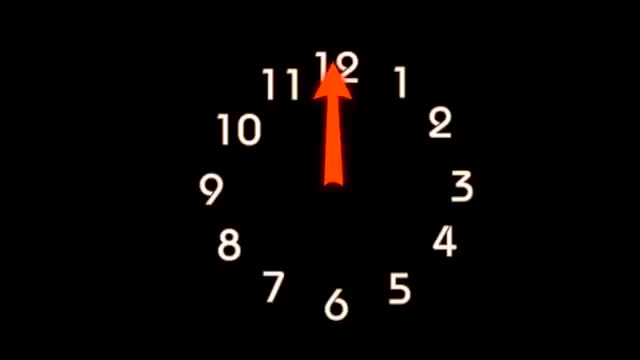The image depicts a minimalist digital clock set against a solid black background. White numerals, ranging from 1 to 12, are arranged in a perfect circle, mimicking the layout of a traditional clock face. A single red-orange arrow points sharply at the 12 o'clock position, indicating the time. The absence of a physical clock frame enhances the digital aesthetic, leaving only the essential elements - the circular arrangement of white numbers and the striking red-orange arrow - clearly visible. The uniform spacing of the numerals in their circular formation underscores the clock's simplicity and precision.